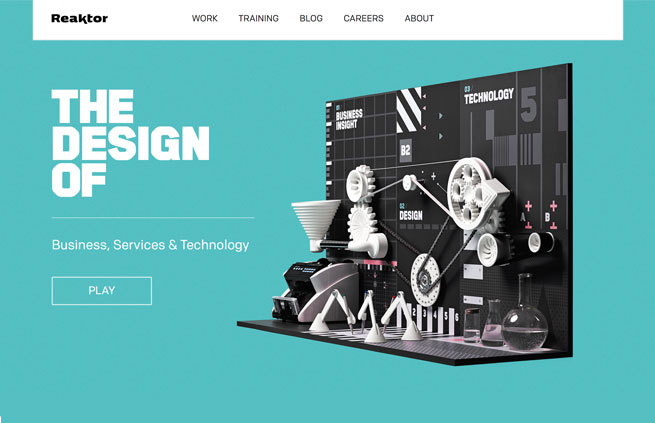The web page image displays the title "Richter" in bold black text, accompanied by navigation options including "Work," "Training," "Log," "Careers," and "About." The main content features text in white that reads "The Design of," with subsections labeled "Business," "Services," and "Technology." A prominent white play button is also visible. The page's background showcases a light blue, aqua-toned hue.

Central to the imagery is a detailed depiction of a complex machine against a black background. This machine comprises multiple interconnected white gears and various components, evoking the appearance of an intricately assembled device or gadget. Sections of the machine are labeled with terms such as "Business Insight," "Design," and "Technology." Additionally, several bottles partially filled with what appears to be water are integrated into the machine's design, contributing to the overall theme of the page. The visual combination of mechanical elements and text creates an impression of a sophisticated, technology-driven interface.